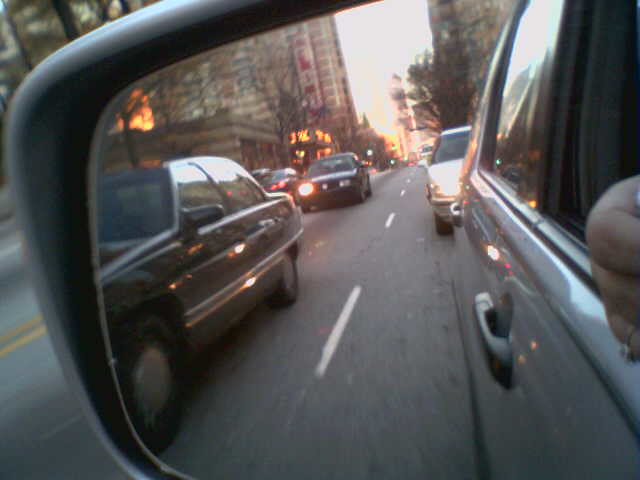This photograph captures a detailed street view from inside a car, focused prominently on the rear-view mirror. The mirror, with its gray edge, spans diagonally from the top middle right to the lower left of the image, revealing a silver car with a closed hand hanging out of the window. In the mirror's reflection, a white car with its headlights on follows closely, while a black car with one headlight functional trails behind it. Further to the left, a darker Cadillac-like vehicle is visible, partially distorted. The concrete road with a white dotted line runs down the center, flanked on the left side by a row of trees that have lost their leaves. Tall buildings, including a large, slender one, rise into the sky in the background, with the sun either rising or setting behind them, casting a warm glow.